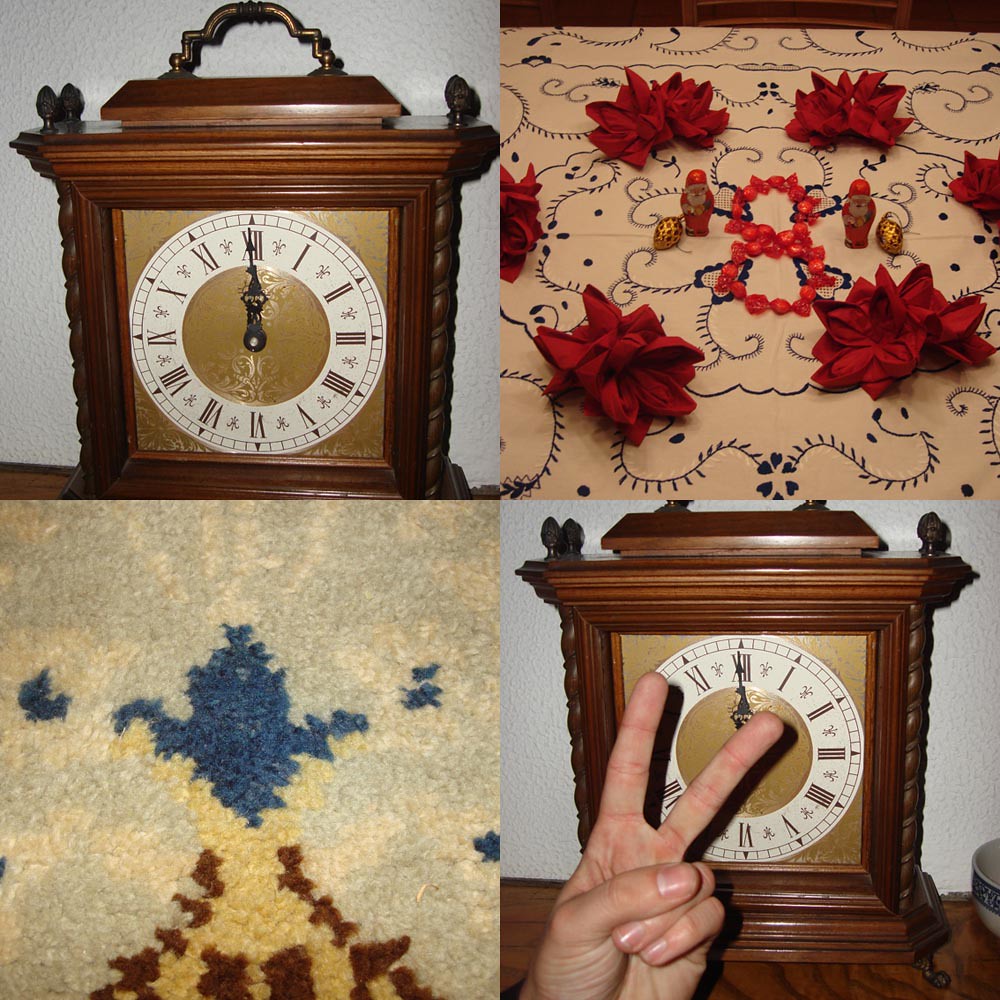The image consists of four distinct pictures arranged in a grid. 

**Top Left:** A vintage-style clock crafted from brown wood, featuring a gleaming gold handle. It resembles a classic grandfather clock with its ornate design. The clock face is encased in a gold square border, while the dial itself forms a round circle adorned with gold Roman numerals. Black minute and hour hands stand out against the shiny gold center, which matches the gold border. The wooden edges are intricately carved, adding a touch of elegance to the overall design.

**Top Right:** A beige tablecloth or decorative fabric with intricate black designs. The centerpiece is composed of six red flowers, resembling Poinsettias, arranged in a circular pattern. Among these flowers are small Santa Claus figures, reminiscent of foil-wrapped chocolate candies. Additionally, there are two gold foil-wrapped items with red accents, possibly chocolate eggs, and a figure-eight formation made from small red objects.

**Bottom Left:** A close-up of a carpet with a beige base featuring a subtle gray tint. The central design is an ornamental emblem in blue and beige, bordered in brown. The intricate pattern contrasts with the carpet's muted background, providing a sense of sophistication.

**Bottom Right:** A repeat of the previously mentioned clock, but this time a hand is visible in the foreground, displaying a peace sign. The hand partially obscures the clock, adding a human element to the image.